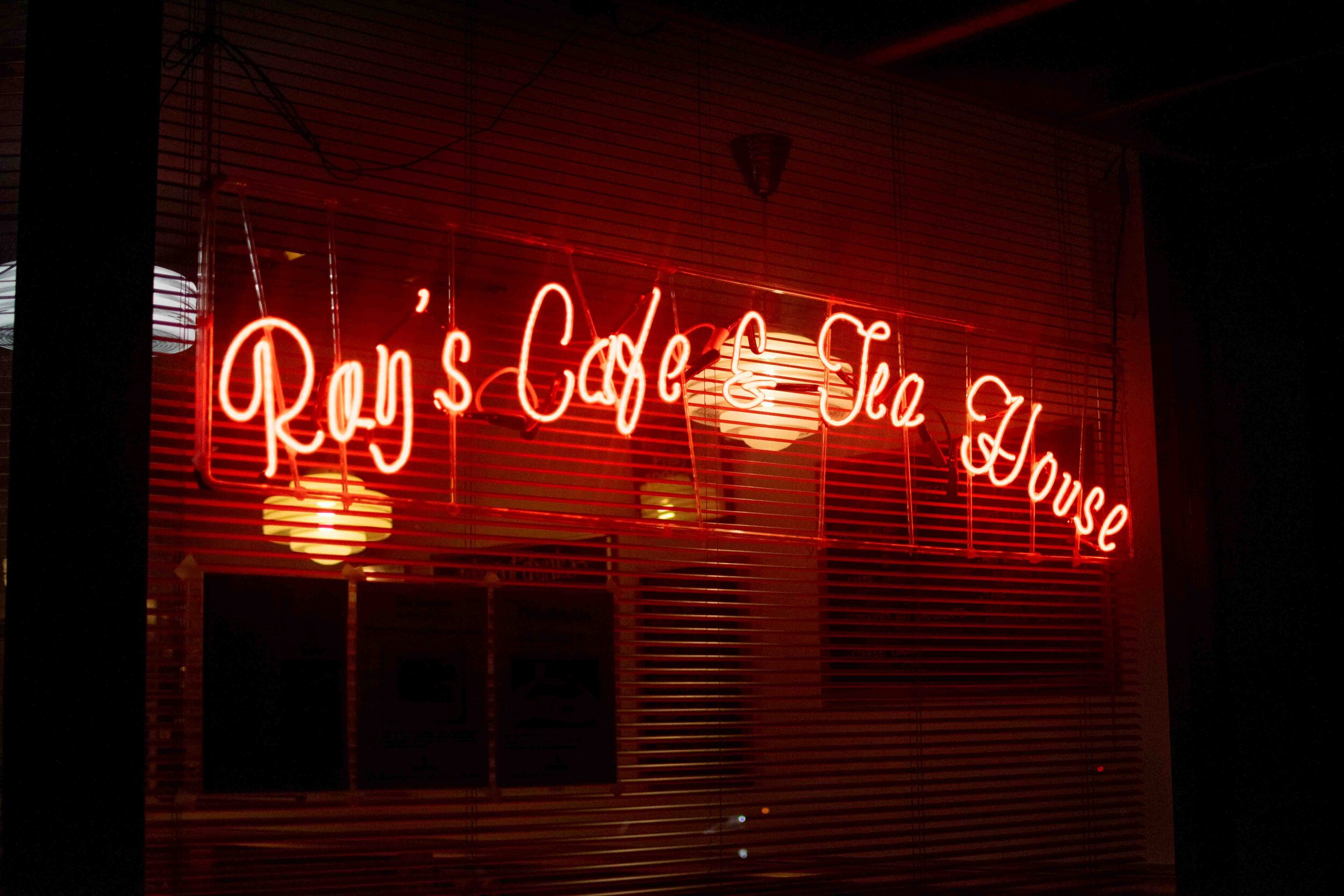The image captures a vibrant neon sign for "Ray's Cafe and Tea House," glowing in bright red cursive lettering. The sign takes center stage against a dark, black background, suggestive of an illuminated evening scene. The curved and nostalgic design of the sign evokes the charm of old-timey diners. 

Located on the window of the establishment, the neon light partially illuminates the surrounding area, giving a glimpse into the interior. Inside, partially open blinds in a darkish orange hue can be seen, alongside hanging lights that would typically be positioned over tables, adding to the cozy ambiance of the tea house. The entire setting around the sign remains shadowed, highlighting the luminescence of the sign and lending a warm, inviting feel to the cafe's facade.